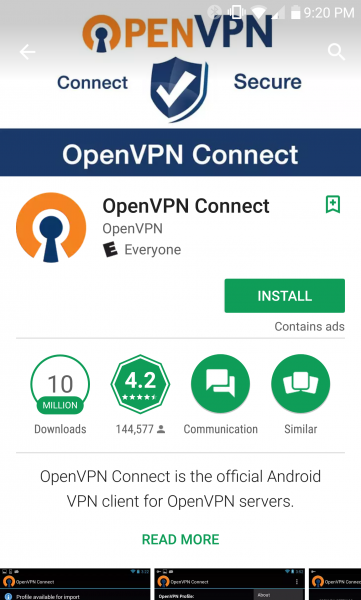This screenshot from a cell phone displays the interface for the OpenVPN application. At the top of the screen, the OpenVPN logo is prominently featured, with the "O" creatively designed to resemble a door lock. Below the logo, two options are available: "Connect" and "Secure." Central to the screen, a large blue shield icon with a white check mark emphasizes security. Further down, a dark blue rectangle spans the width of the screen, displaying the text "OpenVPN Connect" in white letters, signifying a quick link to initiate a connection. A pop-up has appeared, likely after the "OpenVPN Connect" button was clicked, reiterating "OpenVPN Connect" and featuring a green "Install" button for easy installation. Additional options are available below for further configuration.